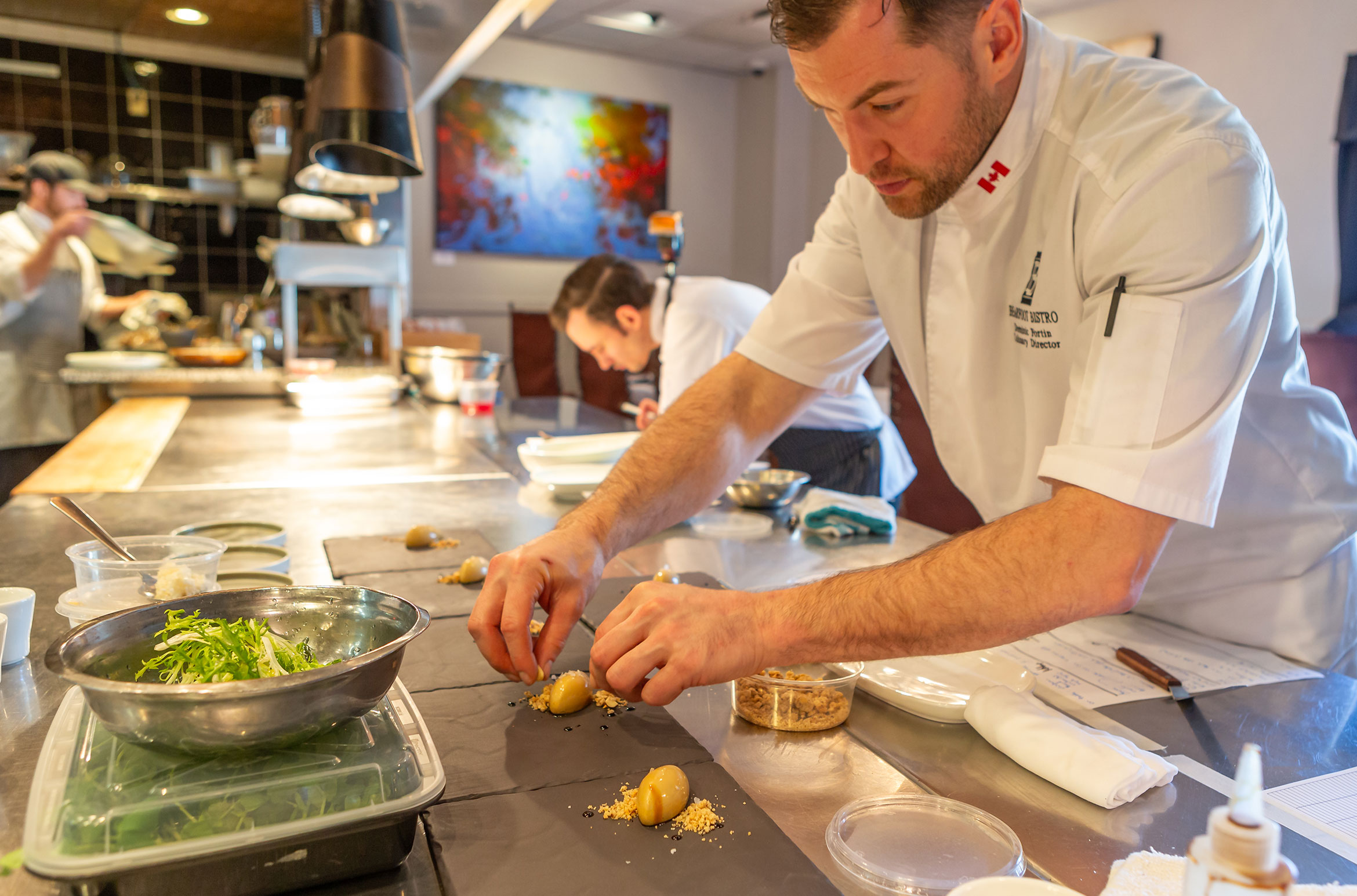In this vivid color photograph, we find ourselves in a clean, modern restaurant kitchen where three chefs are engrossed in their culinary artistry. At the center of the image, a chef dressed in a white uniform is prominently featured. His short-sleeved jacket has a Canadian flag embroidered on the collar, and an inscription referencing a bistro near his chest. With an intense focus, he plates a sophisticated dish on a series of square slate slabs. Each slab holds a delicate arrangement that includes a yellowish garnish and salad greens. The chef, a Caucasian man, is meticulously adding the final touches, possibly small crumbs, to one of the plates while an orange jelly-like substance decorates the top right corner of each slab.

Behind him, the hustle and bustle of the kitchen continues. One chef, slightly blurred, works diligently at another stainless steel table, while another distant figure, also blurred, appears to be handling a pizza crust. Pendant lights hang from the ceiling, casting a warm illumination over the spotless, stainless-steel work tables that stretch into the background. Additionally, an illuminated map decorates one of the back walls, adding a touch of ambiance to the scene. The attention to detail and the dynamic atmosphere showcase a seamless blend of modernity and culinary tradition.